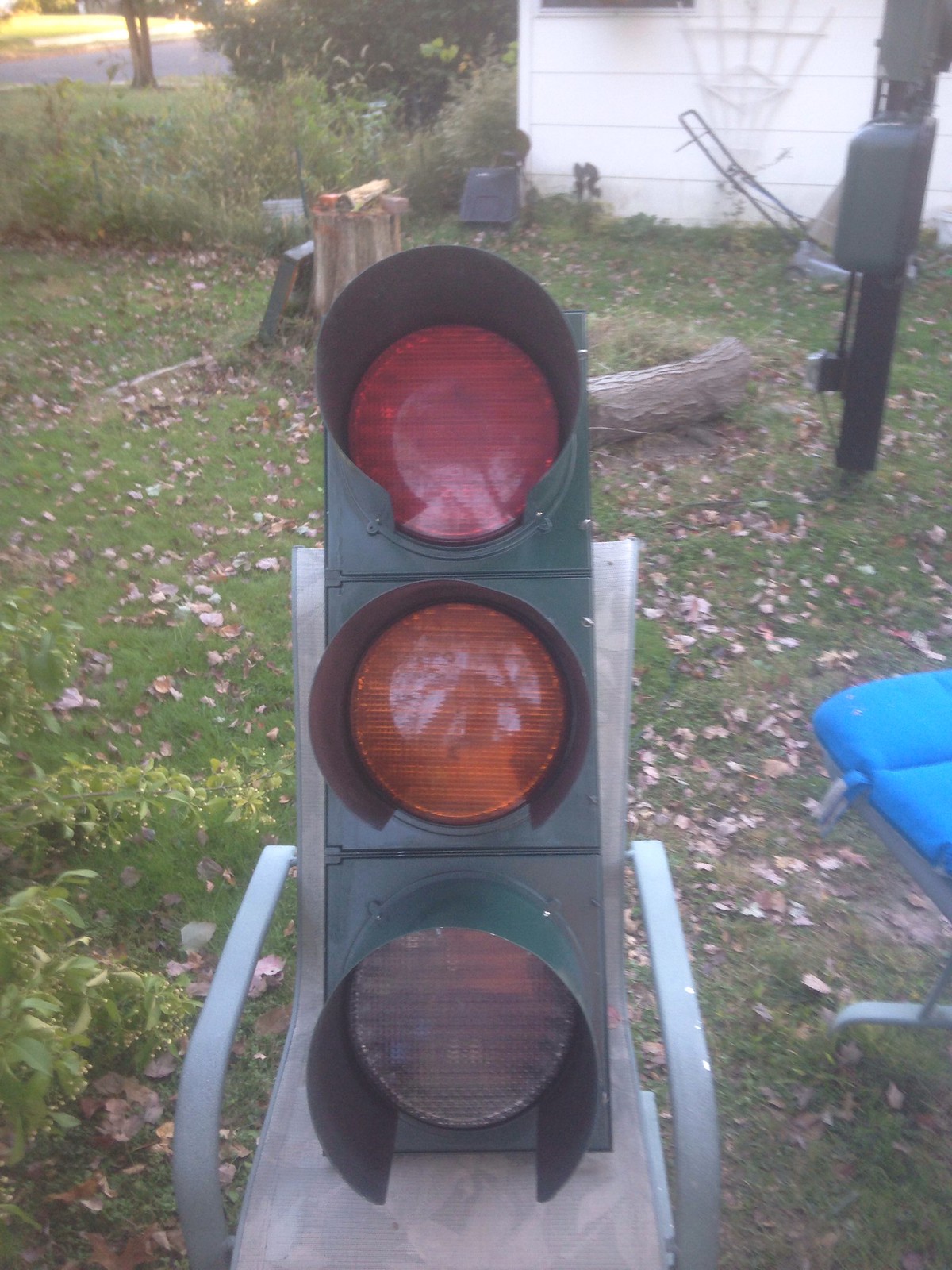In this detailed photograph of a yard, the central focus is a traffic light positioned on a grayish-blue lawn chair. The traffic light, roughly twice the size of the chair, prominently displays a large red light at the top, a large orange light in the middle, and a clear light at the bottom. To the right of this setup is another chair featuring a light blue cushion, partially visible against a gray background. Scattered brownish leaves cover the green grass, which is longer in the background, where a tree stump, a tree trunk, and some logs lie on the ground.

At the upper right corner, there is an intricate black and gray structure consisting of a main supporting section, a gray box, additional black segments, and a protruding black wire. The yard also includes a white house with a trellis, visible in the far back right, along with a black push lawnmower resting against it. The top half of the image shows a stretch of road, various bushes, and part of a tree, all bordered by the long grass and leafy ground cover of this outdoor scene.